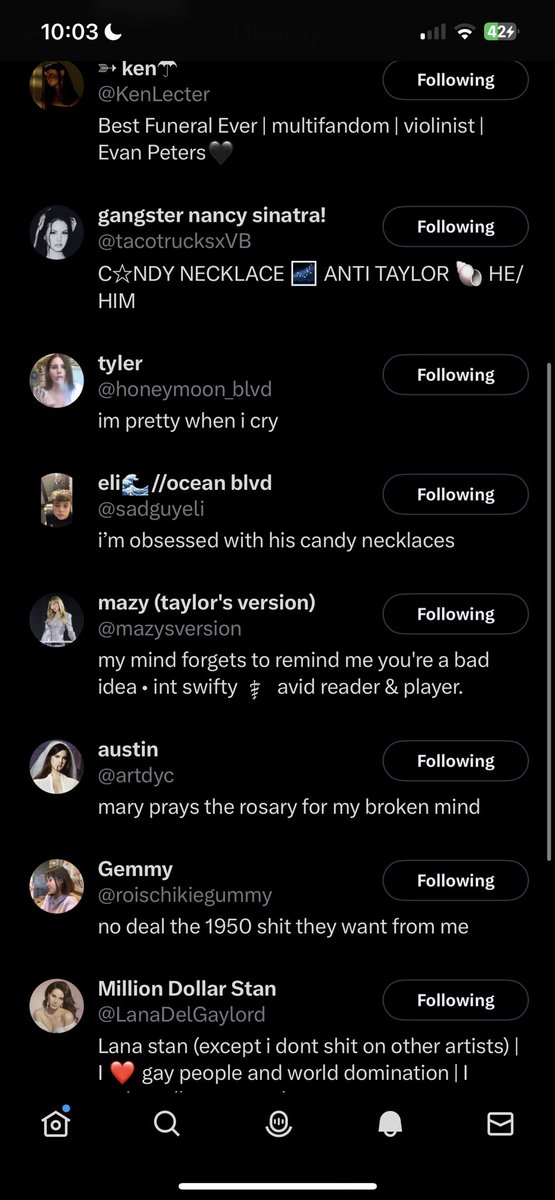The image is a screenshot of notifications from a social media app. The background of the image is entirely black, and at the top, white text displays the current time, "10:03 PM," with a moon icon indicating nighttime. To the right, the screenshot shows poor cell signal strength with only one out of four bars, a Wi-Fi connection icon, and a battery icon indicating 42% battery remaining.

Below this header, the image displays a list of recent notifications from different profiles, all of whom the user is following. Each profile features a distinct custom profile picture, primarily of women, though the gender of a user named Tyler is uncertain.

At the very bottom of the screenshot, there is a navigation bar containing various icons: the home symbol, the search symbol, an unidentified middle icon, the notifications symbol (highlighted as the current page), and another unidentified icon, possibly representing email or sharing options.